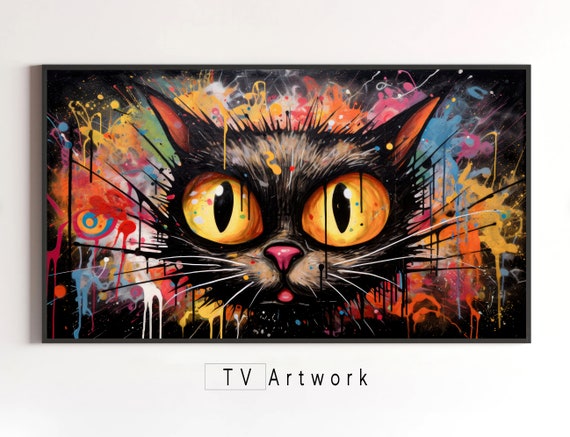This vibrant, horizontal painting features a whimsical black cat with striking, oversized yellow eyes with black pupils. Complementing its playful demeanor, the cat sports a pink nose, a peek of a pink tongue, and spiky whiskers. Its fur, adorned with hints of pink and reddish brown in the ears, appears slightly disheveled, giving it a street cat vibe. The backdrop is a chaotic but vividly colorful explosion reminiscent of fireworks or abstract graffiti, with splotches of orange, yellow, green, blue, pink, purple, and red against a dark black background. Some of these colors even bleed into and drip around the cat, adding to the dynamic feel of the artwork. The image is housed in a thin black frame, mounted on a white wall, with the words "TV artwork" inscribed in black at the bottom.